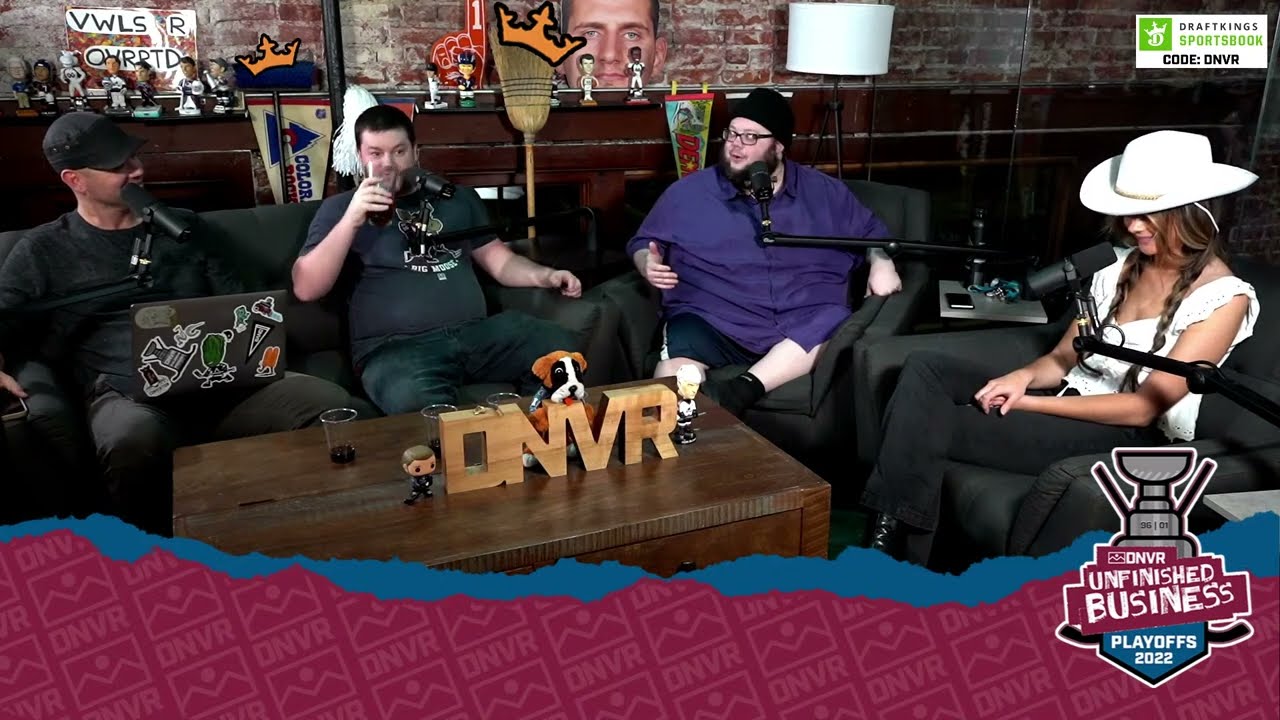The photograph captures a relaxed, conversational setting that appears to be a podcast or radio show recording, most likely related to the Denver sports scene. Four participants are gathered around a dark wooden coffee table, marked with a wooden decoration that reads "DNVR." The table is strewn with a couple of Funko Pop bobbleheads, a stuffed dog, and several drinks, some empty.

Two men are seated on a black loveseat to the left. One man is distinctively featured with a laptop adorned with numerous stickers on his lap. On the right, a woman in a white cowboy hat, white tank top, dark pants, and long braided pigtails sits in a black cushioned chair. Beside her, another man wearing a blue shirt, shorts, and a black hat occupies a similar chair. All individuals are equipped with microphones on black stands, indicative of an ongoing recording session.

The woman is glancing down with a smirk, while two of the men are engaged in conversation, one of whom wears a top hat or fedora. The backdrop features a mix of wood paneling and faux brick with various decorative pennants and additional bobbleheads. Prominently displayed in the top right corner of the image is a sign for "Draft Kings Sportsbook" with the promo code "DNVR," and a poster showing "Unfinished Business, Playoffs 22," hinting at the Stanley Cup, suggesting a Colorado Avalanche podcast.